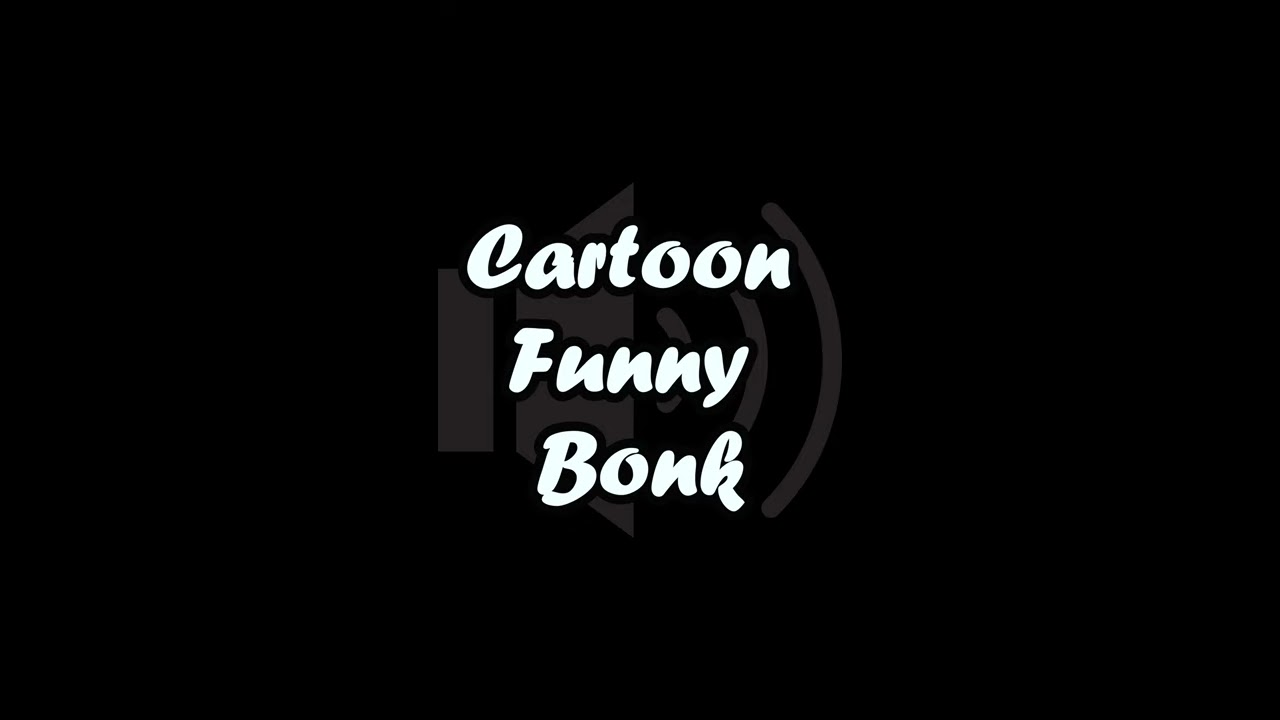This horizontal rectangular image features a minimalist, solid black background with a central focus on text and a symbol. The text is vertically aligned in the center, presented in white bubble letters outlined in black. The words "cartoon," "funny," and "bonk" are stacked on top of each other. Behind this text, there is a semi-transparent dark gray volume symbol. The symbol consists of a vertical rectangle on the left and a trapezoid on its side to the right, from which three increasingly larger curved lines emanate outward. This composition resembles a comic-style title screen with a clear, bold aesthetic.